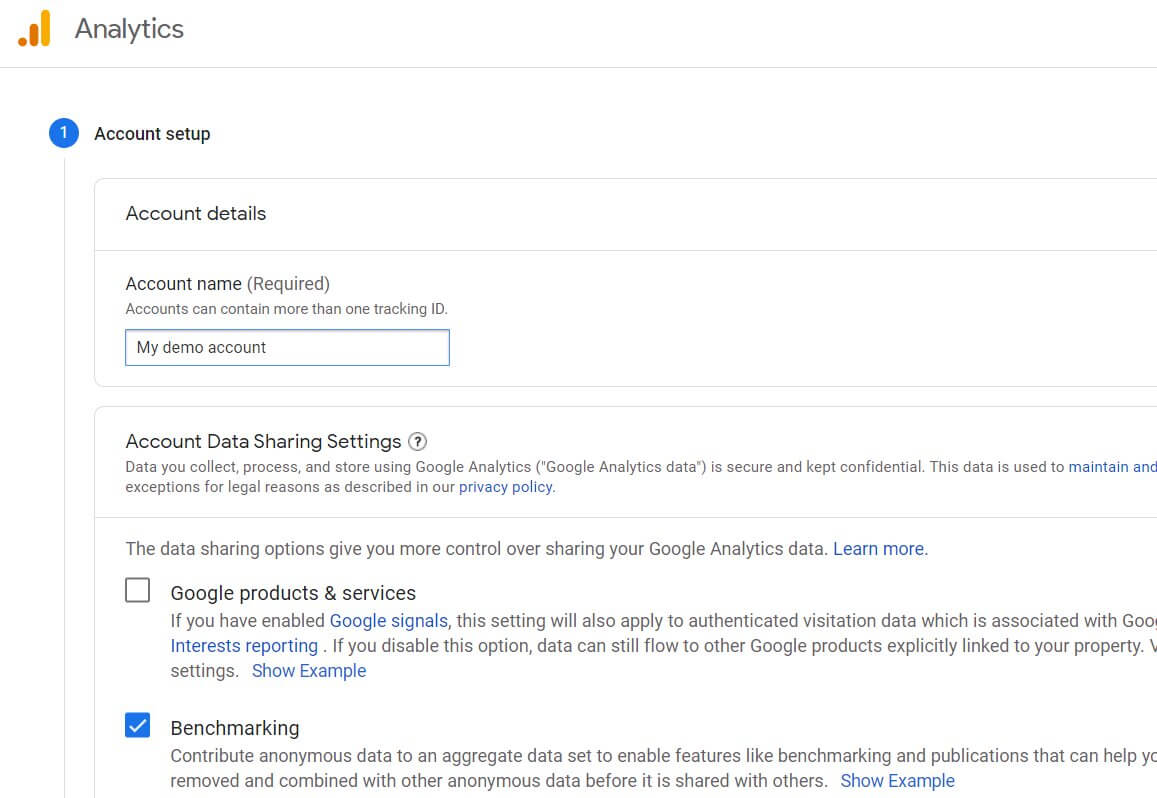This is a detailed caption for an image showing the Google Analytics Account Setup page.

---

The image displays the Account Setup page for Google Analytics, identifiable by the Google Analytics logo in the top left corner, accompanied by the text "Analytics." The page is titled "Account Setup" and is the first step in setting up an account. It prompts the user to enter their account details, with a sample account name filled in as "My Account Demo." A note is present highlighting that accounts can contain more than one tracking ID, implying the presence of unique identifiers for tracking.

Below the account name field, the section titled "Account Data Sharing Settings" is visible, emphasizing the secure and confidential nature of data collected, processed, and stored using Google Analytics. This section includes two checkboxes under the heading "Data Sharing Options," which provide users with choices for sharing their Google Analytics data.

The first checkbox, labeled "Google Products and Services," can be selected to receive email updates about Google products and services. The second checkbox, labeled "Benchmarking," allows users to contribute anonymous data to an aggregate dataset. This dataset enables features such as benchmarking and publications, although part of the text following this description is cut off and cannot be fully read.